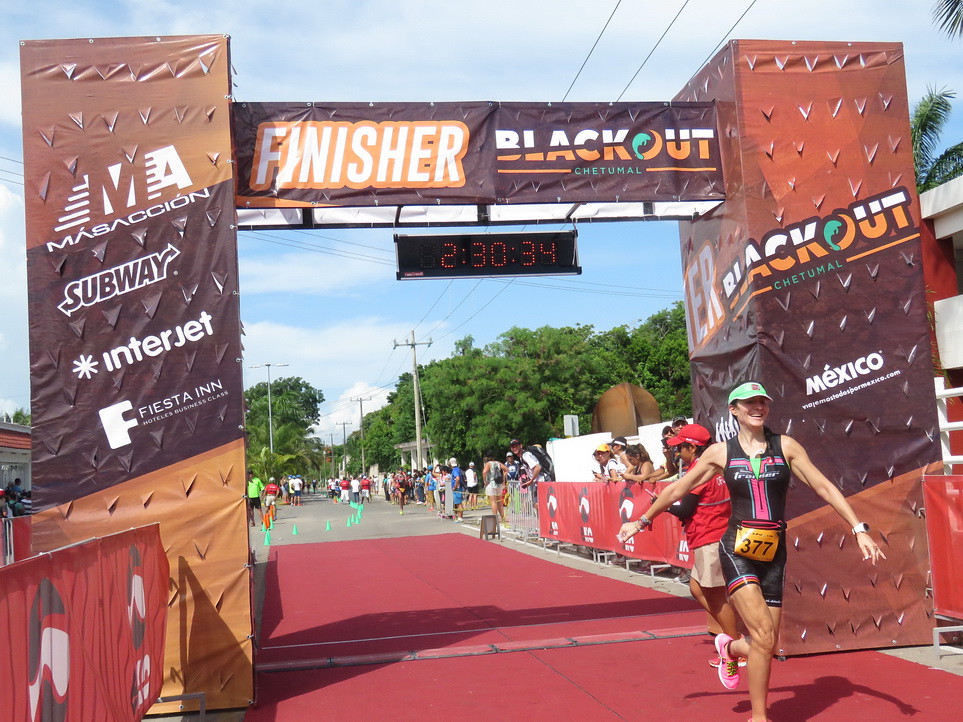This is a full-color photograph capturing the vibrant finish line of a racing event set outdoors on a sunny day with a blue sky and scattered clouds. Central to the image is a young woman, visibly cheerful, who has just crossed the finish line. She wears a black tank top and shorts, both adorned with red and blue detailing, and her outfit is complemented by a blue visor. She proudly displays the number 377 on her hip. 

The finish line itself is marked by a brown gateway structure bearing the words "Finisher, Blackout, Chetumal" in white letters with an orange outline. Just below the sign, a digital display shows the time as 2:30:34 in red digits. The ground beneath this structure is covered in a red carpet, emphasizing the celebratory environment.

Flanking the runner, spectators stand along both sides of the pathway, adding to the scene's lively atmosphere. The backdrop reveals green trees and blue cones, further tying the scene together. Noticeable sponsors such as Subway, Interjet, Fiesta Inn, and Blackout are present, hinting at the event's locale, likely in Mexico. In the background, a man in red, seemingly an official or timekeeper, can be seen ensuring the smooth progression of the race.